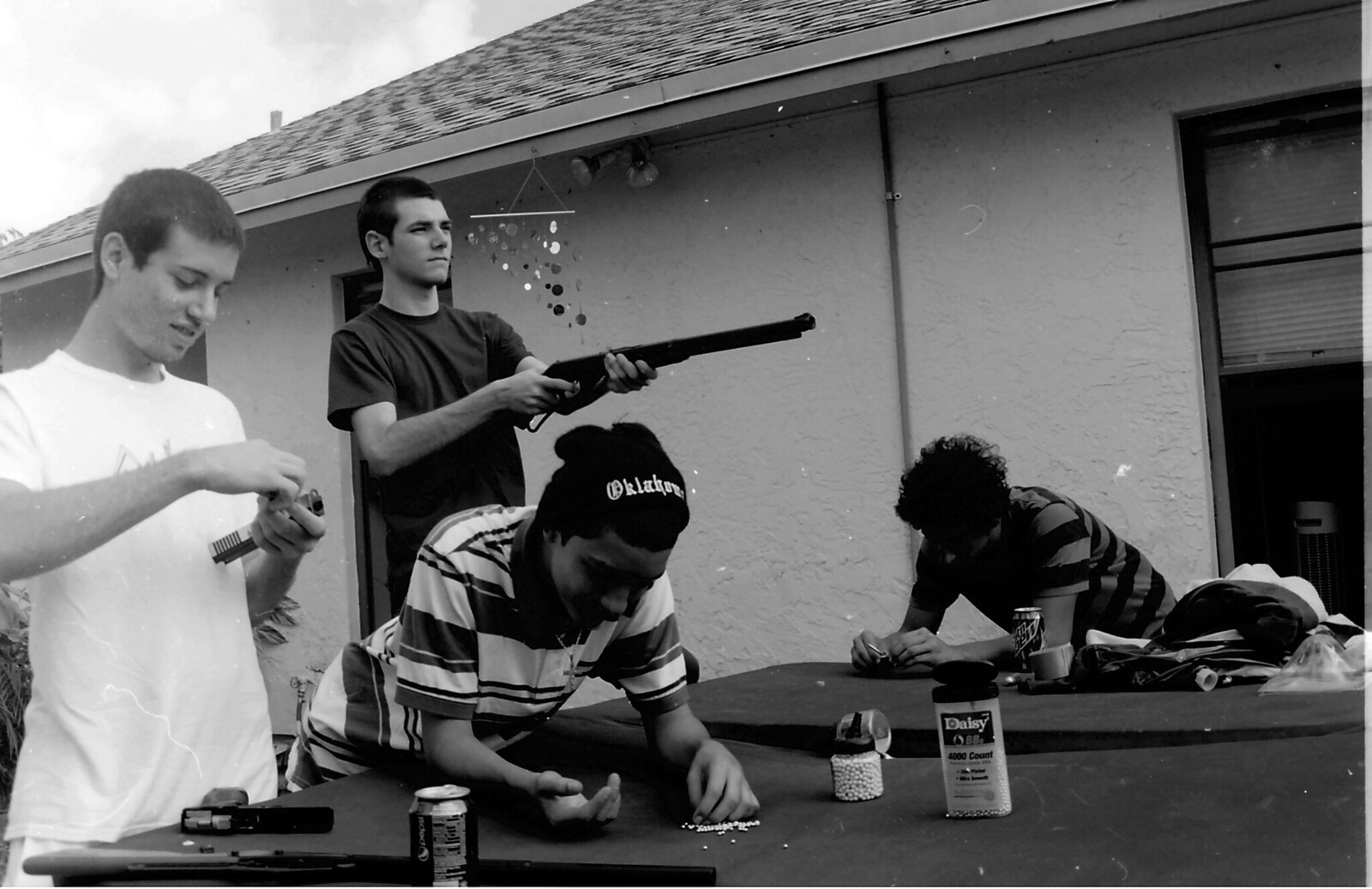In this black-and-white photograph, four young men, possibly in their late teens or early twenties, are gathered outside a typical residential house on a cloudy day. The background shows parts of the house like the roof and a visible window. The men appear to be engaged in an activity involving BB guns and BB pellets. 

On a dark-surfaced table in front of them, there's a container labeled "Daisy" filled with BB pellets. One man, dressed in a white shirt, is intensely focused as he loads a pistol with BBs. Beside him, another man handles a rifle, aiming it into the distance. Two other men, wearing striped shirts, can be seen sorting through the BB pellets on the table, potentially getting ready to load their own BB guns. One of these men also wears a beanie. The detailed setup and the individuals' actions convey a scene of focused preparation and leisure.